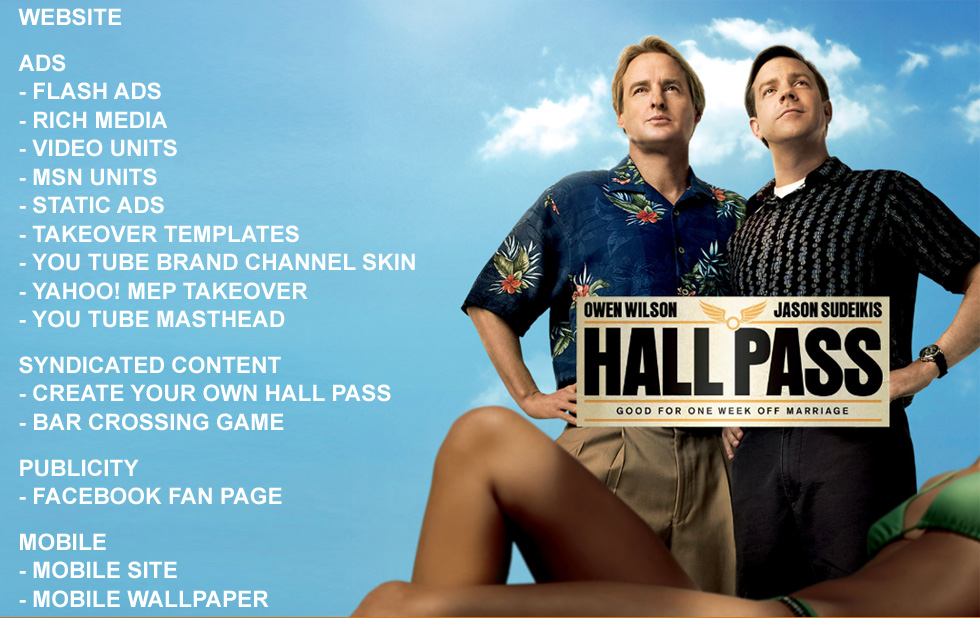The image is an advertisement for the movie *Hall Pass* featuring Owen Wilson and Jason Sudeikis. The primary focus of the image is on the two main actors, who are standing closely together with their hands on their hips, gazing into the distance. They are dressed in casual attire: Owen Wilson dons a blue orchid print shirt with tan pants, while Jason Sudeikis wears darker clothing. The background features a blue sky with some white clouds. In front of the actors, partially out of frame, is a woman in a green bikini, emphasizing her legs and abdomen.

The right side of the image prominently displays the movie's title *Hall Pass: Good for One Week Off Marriage* in a yellowish-gold rectangle with black font. The left side of the image contains a vertical column of white text listing various marketing and advertising components, such as "Website, Ads, Flash Ads, Rich Media, Video Units, MSN Units, Static Ads, Takeover Templates, YouTube Brand Channel Skin, Yahoo MEP Takeover, YouTube Masthead," among others. These details suggest that the image may be part of a broader marketing and promotional strategy aimed at advertisers and marketers.